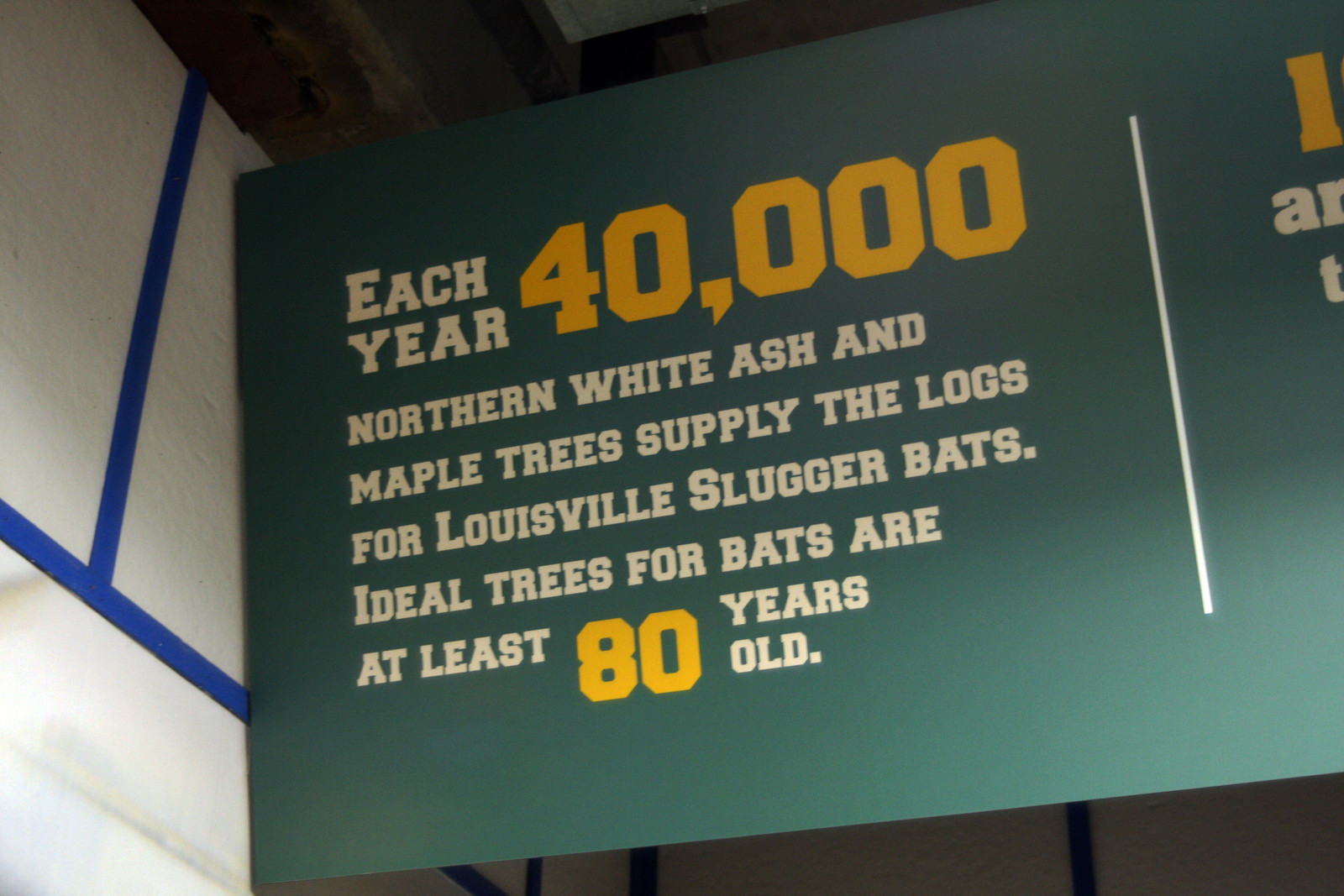This color photograph is a close-up of an informational sign with a dark green background, white letters, and highlighted numbers in orange. The sign reads, "Each year 40,000 northern white ash and maple trees supply the logs for Louisville Slugger bats. Ideal trees for bats are at least 80 years old." The photograph cuts off part of the sign, limiting visibility to this specific section. The sign appears to be positioned higher than the camera, suggesting an upwards angle. It is affixed against a white wall with blue trim, and there's a wooden ceiling above. Additionally, a foam board with two lines of duct tape is visible next to the sign. There are no other discernible objects in the background.